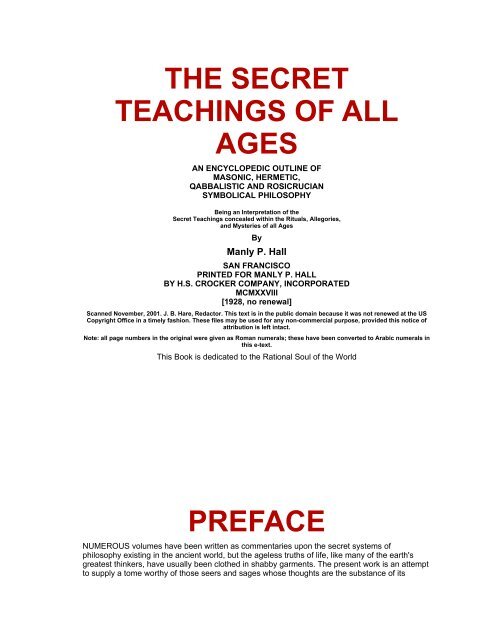This is an image of a detailed text from a book cover or page. At the top, in red letters, it reads, "The Secret Teachings of All Ages." Below, in black, it states, "An encyclopedic outline of Masonic, Hermetic, Qabbalistic, and Rosicrucian Symbolical Philosophy," followed by "Being an interpretation of the secret teachings concealed within the rituals, allegories, and mysteries of all ages." The author is Manly P. Hall, and the book was printed in San Francisco for Manly P. Hall by H.S. Crocker Company, Inc., in 1928, with no renewal. There is some additional smaller and harder-to-read text. The book is dedicated "to the rational soul of the world." Following the dedication, there is a preface which begins with, "Numerous volumes have been written as commentaries upon the secret systems of philosophy existing in the ancient world, but the ageless truths of life, like many of the earth's greatest thinkers, have usually been clothed in shabby garments. The present work is an attempt to supply a tome worthy of those seers and sages whose thoughts are the substance of its..."